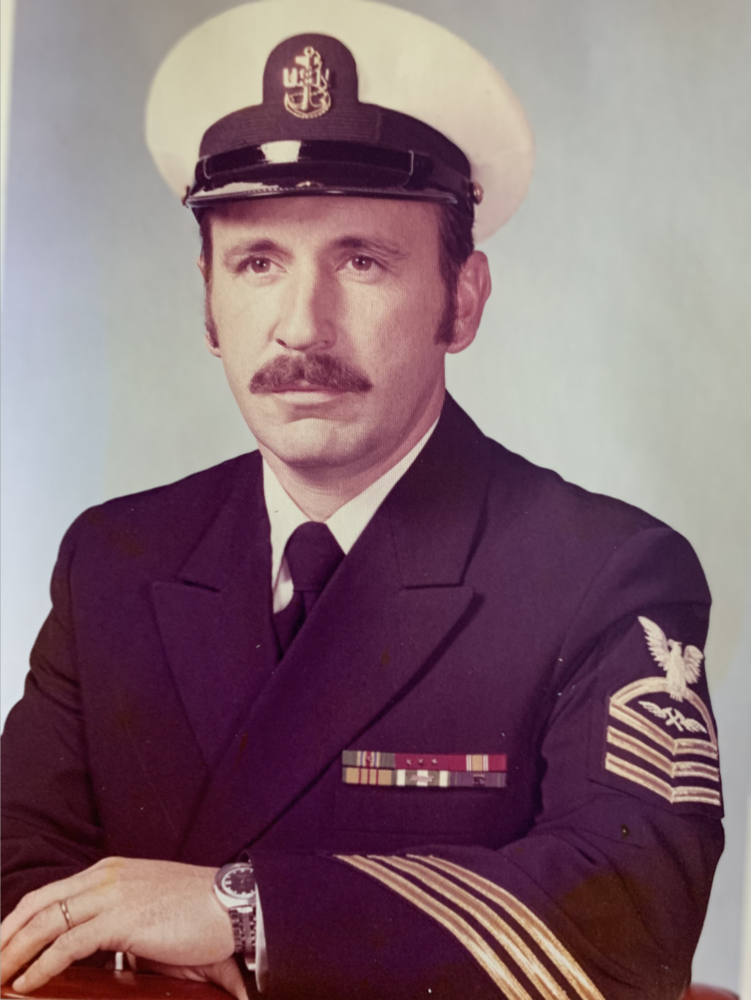The image is a faded, grainy vintage photograph of a middle-aged man posed for a portrait, likely from the 1980s. He appears to be a high-ranking military official, possibly a captain or admiral, indicated by his decorated uniform. He is dressed in a dark black jacket adorned with badges and medals above his left breast pocket, a black tie, and a white collared shirt. A silver watch is visible on his wrist. His uniform is detailed with a crest on his shoulder pad that resembles an eagle with outstretched wings and additional golden embellishments. He sports a white captain's cap with a black brim, featuring a symbol at its center. The man has a moustache and is looking directly ahead, embodying a distinguished and authoritative presence.